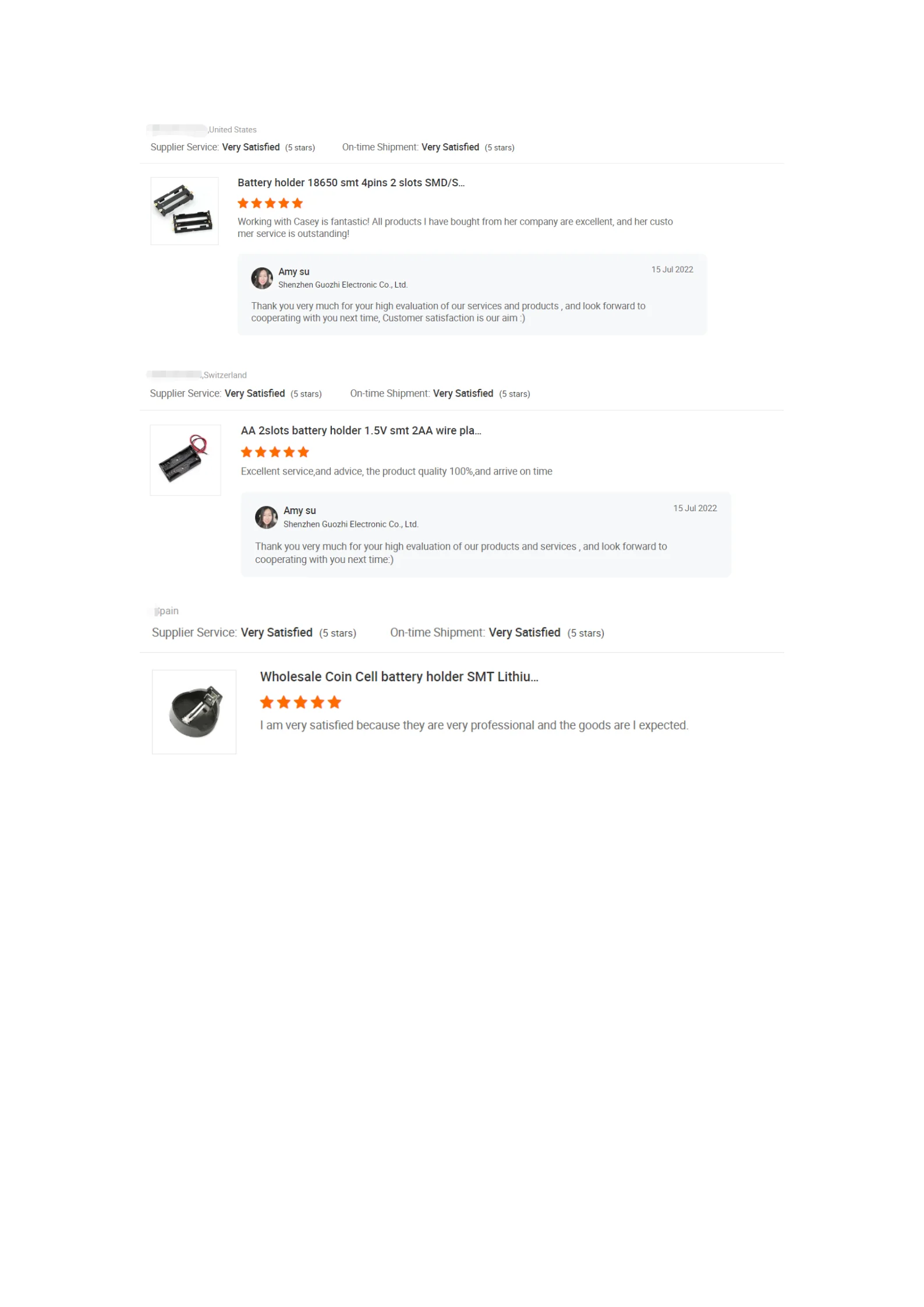**Detailed Caption:**

The image displays a series of three customer reviews for electronic products, presented in a structured format. Each review is formatted consistently, starting with the country of origin, "United States," which has some parts of the address blurred for privacy.

### Review 1:
- **Service Quality**: Supply service and on-time shipment rated as "Very Satisfied" with five stars each.
- **Product**: Battery holder, 18650, SMT, four pins, two slots.
- **Rating**: Five orange stars.
- **Comment**: "Working with Casey is fantastic, all products I have bought from her company are excellent, and her customer service is outstanding."
- **Response**: From Amy Su of Xin Xin Guzi Electronic Company, dated July 15, 2022, expressed gratitude for the customer's high evaluation and looked forward to future cooperation, emphasizing customer satisfaction as their aim.

### Review 2:
- **Service Quality**: Both supply service and on-time shipment rated as "Very Satisfied" with five stars each.
- **Product**: Clearly indicated as another electronic component.
- **Rating**: Five orange stars.
- **Response**: From Amy Su reiterating the same level of gratitude and enthusiasm for future cooperation, similar to the first response.

### Review 3:
- **Service Quality**: Both supply service and on-time shipment rated as "Very Satisfied" with five stars each.
- **Product**: Wholesale coin cell battery, SMT, lithium (title is truncated).
- **Rating**: Five orange stars.
- **Comment**: Not fully displayed in the given excerpt.
- **Response**: Indicated but not detailed in the given excerpt, presumed to be similar in tone and content as the previous responses. 

Each review highlights a detailed appreciation for the product quality and exceptional customer service, with consistent positive feedback from the customers and cordial acknowledgments from Amy Su of Xin Xin Guzi Electronic Company.